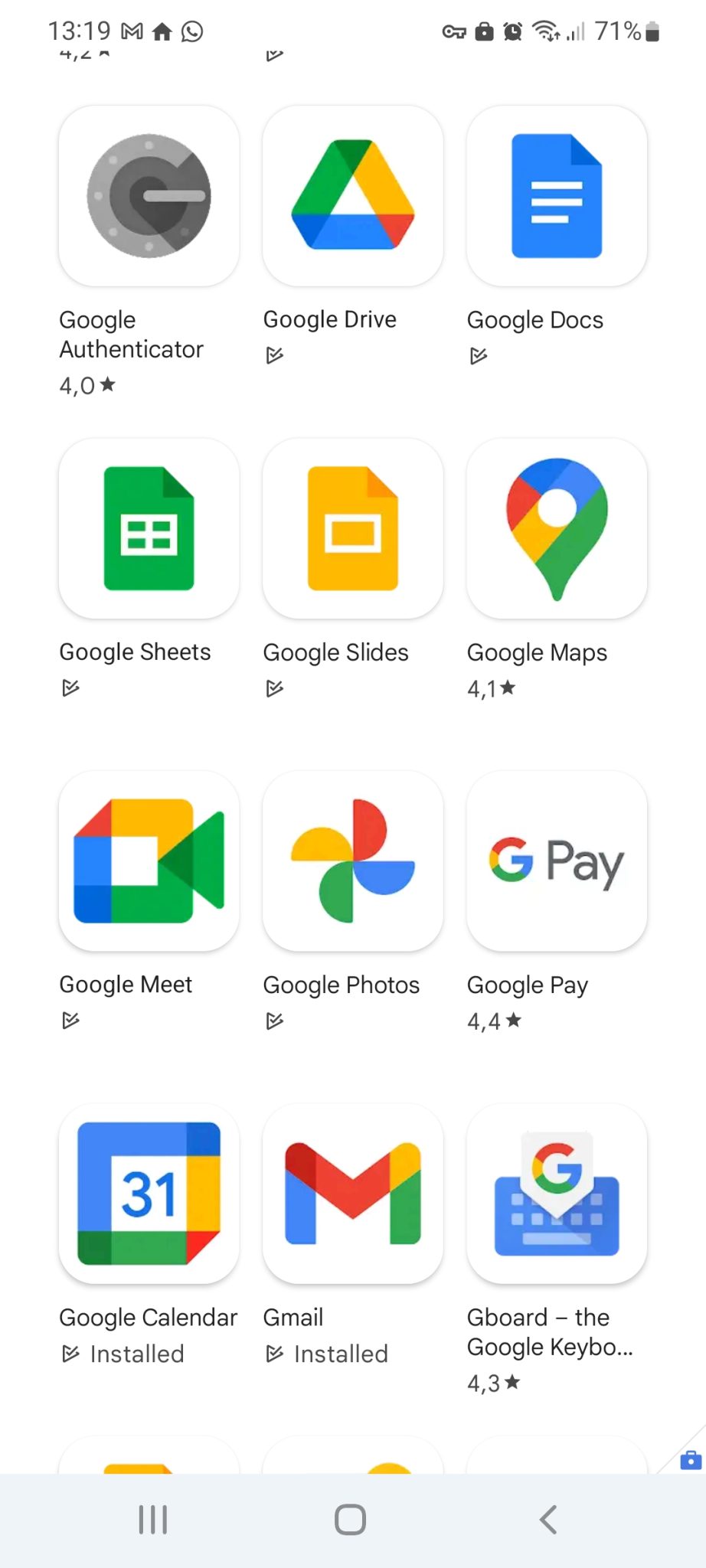The image is a vertical screenshot, likely taken from a smartphone. The background is plain white, possibly rendered from the screen it's displayed on. At the very top left corner, the time is shown as 13:19 in military format, alongside various icons including "M," "Home Screen," and another unspecified one. The top right corner features a series of icons: a key and padlock, an alarm clock, Wi-Fi signal, cellular signal strength, and a battery icon indicating 71% charge.

The main focus of the image comprises a grid layout of app icons arranged in three columns and four rows, all with rounded edges. Each icon displays the app's name beneath it. The visible apps are:

1. Google Authenticator (with a rating of 4.0 stars)
2. Google Drive
3. Google Docs
4. Google Sheets
5. Google Slides
6. Google Maps (with a rating of 4.1 stars)
7. Google Meet
8. Google Photos
9. Google Pay (with a rating of 4.4 stars)
10. Google Calendar (marked as "installed")
11. Gmail (marked as "installed")
12. Gboard - the Google keyboard (with a rating of 4.3 stars)

Additionally, there are other icons visible at the bottom of the screen, likely shortcuts to essential apps or functions on the smartphone.